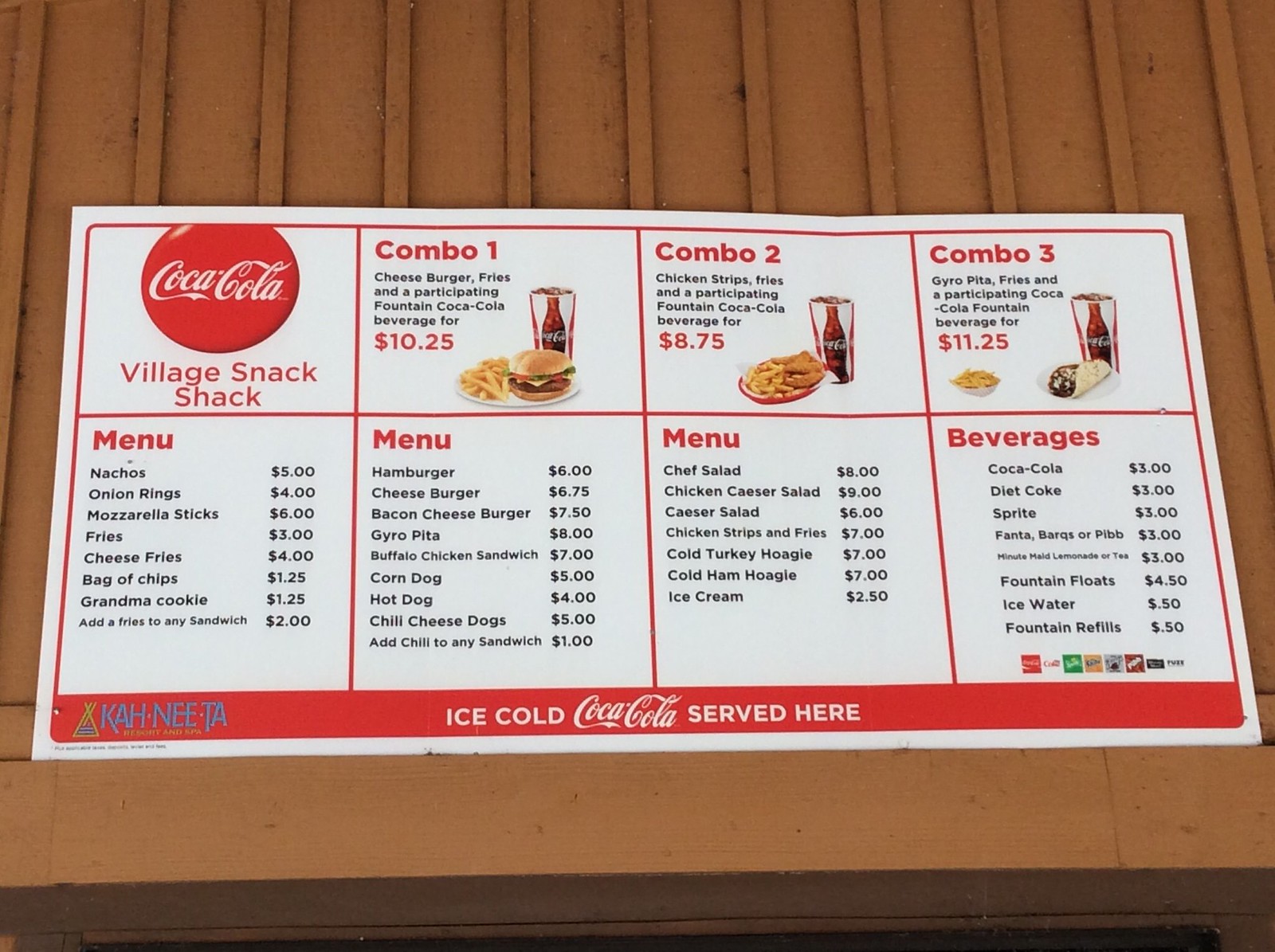This image features a menu from the Village Snack Shack, prominently branded as a Coca-Cola advertisement. The menu appears to be printed on a piece of stiff cardboard, potentially doubling as a placemat. It is shown leaning against a metallic surface resembling a metal roof, suggesting an indoor setting. 

The menu is brown with a large Coca-Cola logo at the top left corner, the most eye-catching element on the page. Below the menu, there is a bright red banner with the text "Ice Cold Coca-Cola Served Here," in Coca-Cola's iconic script. This banner also references Kanita Hot Springs.

The menu is straightforward and diner-style, listing combos and individual items. At the top, it displays combo options labeled as Combo 1, Combo 2, and Combo 3, each including a paper cup featuring a Coca-Cola image. Below, the menu is divided into sections: "Menu," and "Beverages." The "Menu" section lists items like chef salad, chicken Caesar salad, Caesar salad, hamburgers, cheeseburgers, nachos, onion rings, and mozzarella sticks, alongside various combinations of these items. 

Overall, the image captures a nostalgic and simple dining experience, emphasizing the classic pairing of diner food with a refreshing Coca-Cola.